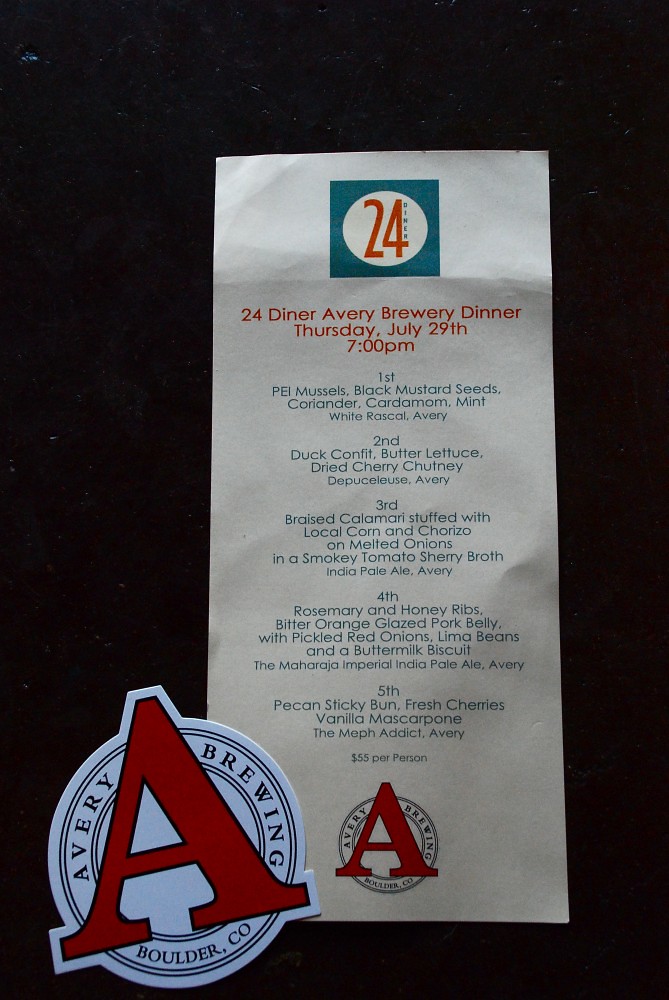The image depicts a detailed brochure for the "24 Diner Avery Brewery Dinner" scheduled for Thursday, July 29th, at 7 p.m. At the top, there's a distinctive logo featuring a blue square with a white circle, inside of which the red numbers "24" and the word "diner" in small black letters are inscribed. The dinner is a five-course meal described meticulously:

1. **First Course**: PEI Mussels adorned with Black Mustard Seeds, Coriander, Cardamom, Mint, paired with White Rascal Avery.
2. **Second Course**: Duck Confit served with Butter Lettuce and Dried Cherry Chutney, complemented by Duplisk Avery.
3. **Third Course**: Braised Calamari stuffed with local corn and chorizo, laid on a bed of melted onions in a Smoky Tomato Sherry Broth, accompanied by an Indian Pale Ale.
4. **Fourth Course**: Rosemary and Honey Ribs with Bitter Orange Glazed Pork Belly, garnished with Pickled Red Onions, Lima Beans, and served with a Buttermilk Biscuit.
5. **Fifth Course**: Pecan Sticky Bun with Fresh Cherries and Vanilla Mascarpone.

The cost per person is noted as $55. Additionally, a larger version of the Avery Brewery logo is visible on the bottom left, featuring a red letter "A" within a circle, encircled by the words "Avery Brewing" and "Boulder, CO." The brochure itself appears to be held up against a black background, possibly by a sticker displaying the same Avery Brewing logo.